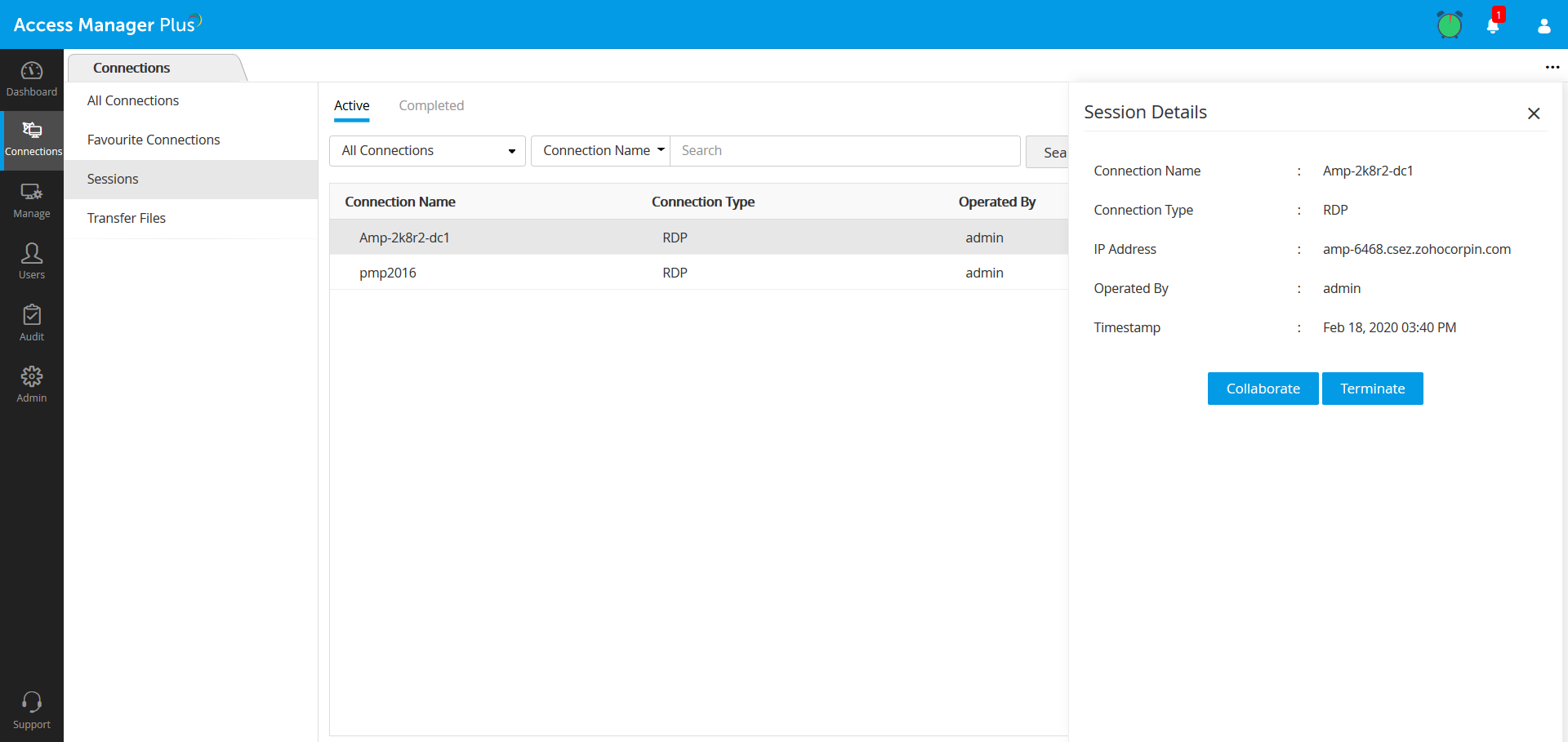Detailed Screenshot Caption:

This screenshot showcases a page from Access Manager Plus. At the top of the screen, the notification bar prominently displays "Access Manager" in bold white text. On the right-hand side, the bar contains three symbols: a green alarm clock, a white bell icon with a red notification bubble marked with the number 1, and an outline of a person in white.

On the left side of the page, there is a vertical menu set against a black background. The menu options listed in light gray text include Dashboard, Connections, Manage, Users, Audit, and Admin. At the bottom of this menu is a support option, represented by a headset icon, also in light gray. 

The "Connections" option has been selected, indicated by a blue vertical line running the entire height of the menu column and the word "Connections" highlighted in white. Under this, a submenu appears with further options: All Connections, Favorite Connections, Sessions, and Transfer Files. The "Sessions" option is highlighted in light gray, denoting it as the active selection. Within the Sessions tab, there are two sub-tabs labeled "Active" and "Completed." The "Active" tab is in black text with a blue underline, indicating it is currently selected, while the "Completed" tab is shown in light gray.

Below this section are dropdowns for filtering sessions by "All Connections" or "Connection Name," followed by a search bar and a search button on the right. The main content area displays session details for the first connection, identified as "AMP-2K8R2-DC1." The specifics include the connection type (RDP), the IP address, the operator, and the timestamp. At the bottom of this section, there are two action buttons titled "Collaborate" and "Terminate," both filled with a light blue color and featuring white text.